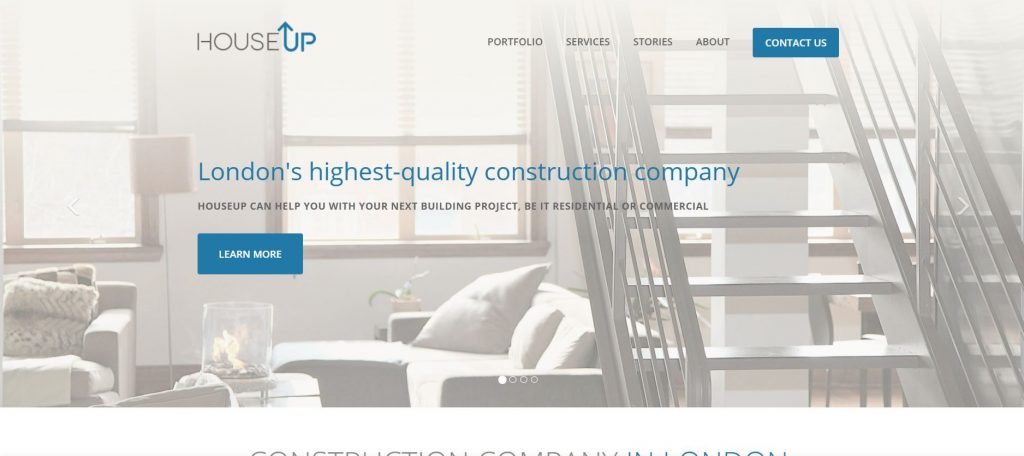This screenshot showcases the homepage of the website "House Up," a premier construction company based in London. The website's title, prominently displayed in the top left corner, features the words "House" in a sophisticated grey-black font and "Up" in a vivid blue font, with the letter "U" stylized as an upward-pointing arrow. 

The top navigation bar offers several clickable options: Portfolio, Services, Stories, About, and Contact Us, with the "Contact Us" button highlighted in a striking blue box. 

Dominating the central section of the screen is a bold headline in blue font proclaiming, "London's Highest Quality Construction Company." Directly beneath, a grey-font subheading elaborates, "House Up can help you with your next building project, be it residential or commercial." Below this text, a blue rectangular button labeled "Learn More" invites visitors to explore the company further.

The background image, slightly out of focus with a delicate faded effect, captures the interior of a house. It depicts a cozy living room on the left side, furnished with sofas, a lamp, and a potted plant on a desk, while windows allow natural light to flood the space. A staircase ascends along the right side of the image, adding a sense of depth and homey ambiance to the overall visual.